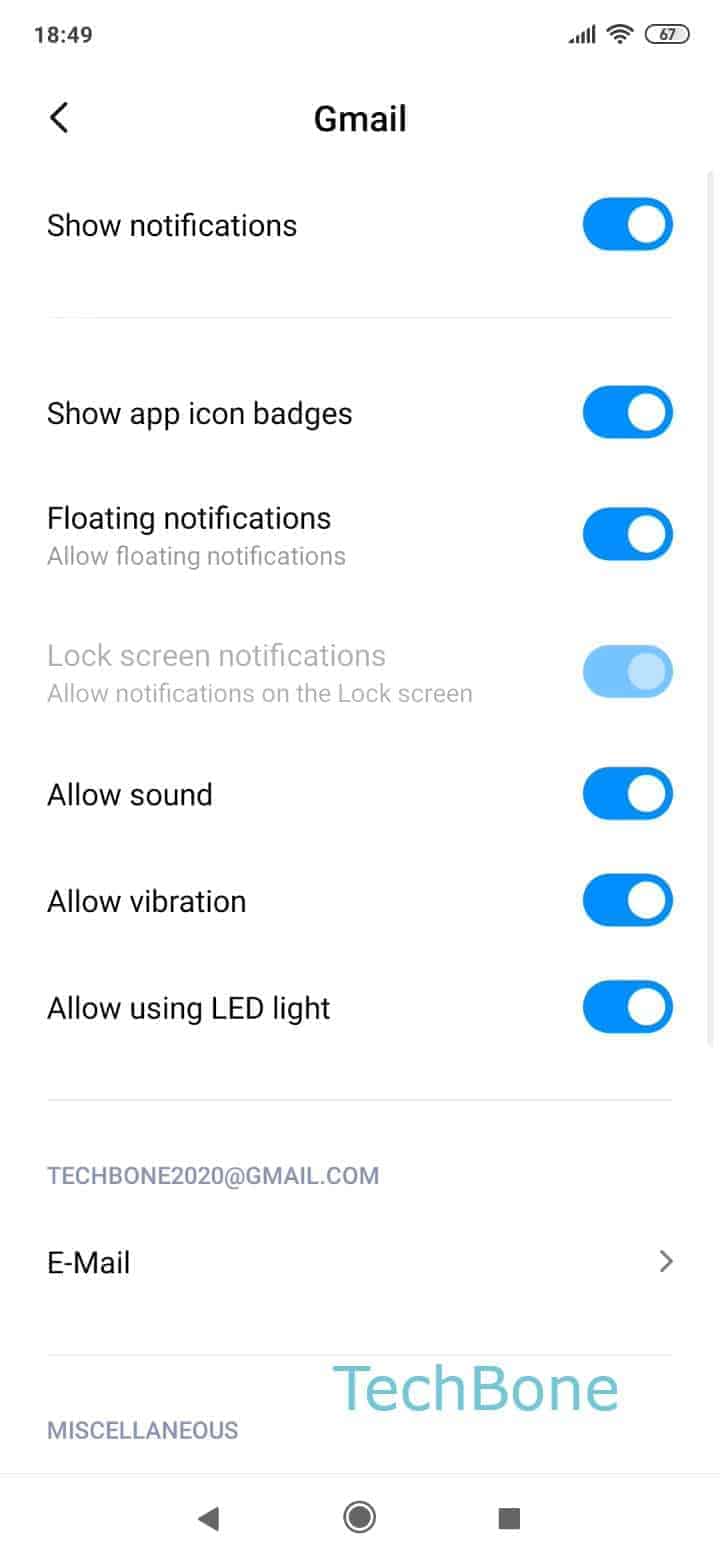The image is a vertical screenshot taken from a smartphone device, displaying a settings page. The background predominantly features a warm off-white or light-yellow hue, contrasting lightly with a gray line running vertically along the right edge.

In the upper left corner, the time is shown as "18:49" in military format. Opposite the time, on the upper right corner, the status indicators include the signal strength bar, the Wi-Fi icon, and a battery percentage reading of 67%.

The top section of the screen has a left-pointing arrow and the label "Gmail," indicating the settings pertain to the Gmail app. Directly below, the option "Show notifications" is visible with a blue toggle indicating it is activated. A series of notification settings follow:

- "App icon badges" with a blue toggle activated.
- "Floating notifications" is also enabled as indicated by the blue toggle.
- "Lock screen notifications" are turned off, as its toggle is not activated.
- "Allow sound" with a blue toggle indicating it is on.
- "Allow vibration" also has its blue toggle on.
- "Allow using LED light" again with an active blue toggle.

Towards the bottom of the screenshot, in gray text, the primary email associated with the settings is displayed as "tech bone 2020 at gmail.com". Below this line, labeled "Email," is an arrow pointing to the right.

Further down, a thin gray line marks a section labeled "Miscellaneous," followed by a prominent, teal-green colored text "tech bone."

At the very bottom of the screenshot is a navigation bar, featuring a left-pointing arrow, a circular record button, and a square button on the right.